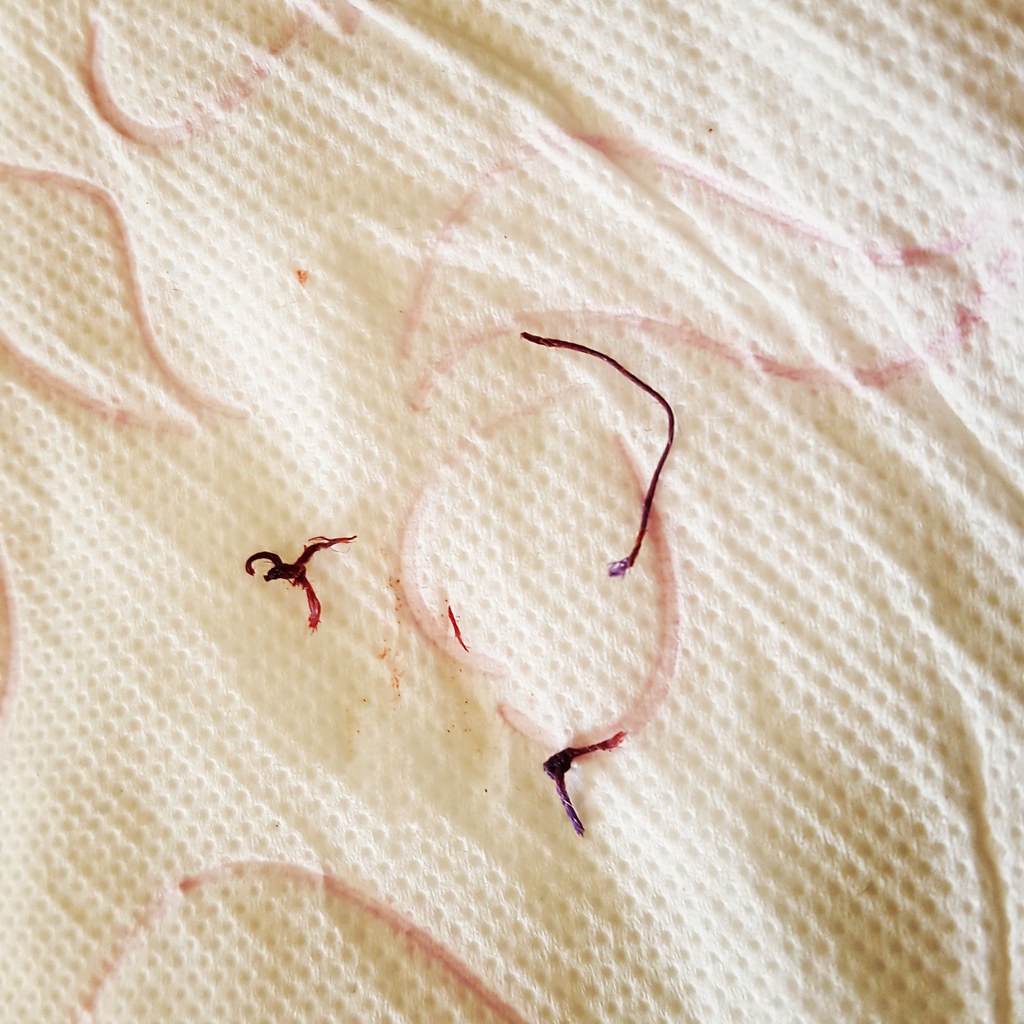The image depicts a highly magnified, close-up view looking directly down onto a textured, off-white paper towel or cloth, resembling a quilt pattern with pilted, circular bumps. Scattered across the surface are several pieces of dark and light red, almost purple, threads. These threads vary in placement and form, with some appearing almost worm-like as they poke up from beneath the textured surface, while others are splatted or frayed on top. In the center, the threads form a knot with three strands extending outward. To the right, there's a shorter, frayed piece and a curved thread about three inches long with its ends pointing leftwards. This detailed zoom showcases the intricate texture and the peculiar arrangement of the threads, giving it an abstract, almost organic quality.